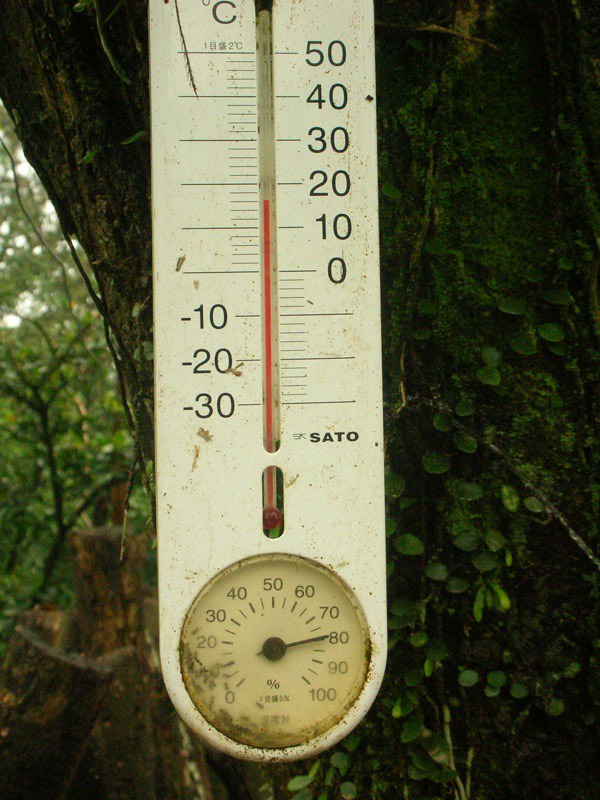The photograph captures a detailed view of a thermometer hanging from the thick trunk of a tree, set against the backdrop of a lush forest or jungle. The tree trunk itself is robust, adorned with small plants and a generous layer of moss, suggesting a humid environment. The thermometer, which is vertical and oblong, displays temperature measurements in Celsius, ranging from -30°C to 50°C. It features a white background that is slightly discolored with rust and dirt specks, indicative of prolonged exposure to the elements.

At the bottom of the thermometer, a circular dial, encased in clear plastic, shows readings from 0 to 100. The dial hand points to 80, and the dial is further embellished with Chinese characters. The photograph is taken during the daytime, allowing the natural light to illuminate the intricate details of the scene, from the texture of the tree bark to the minute dirt particles on the thermometer.